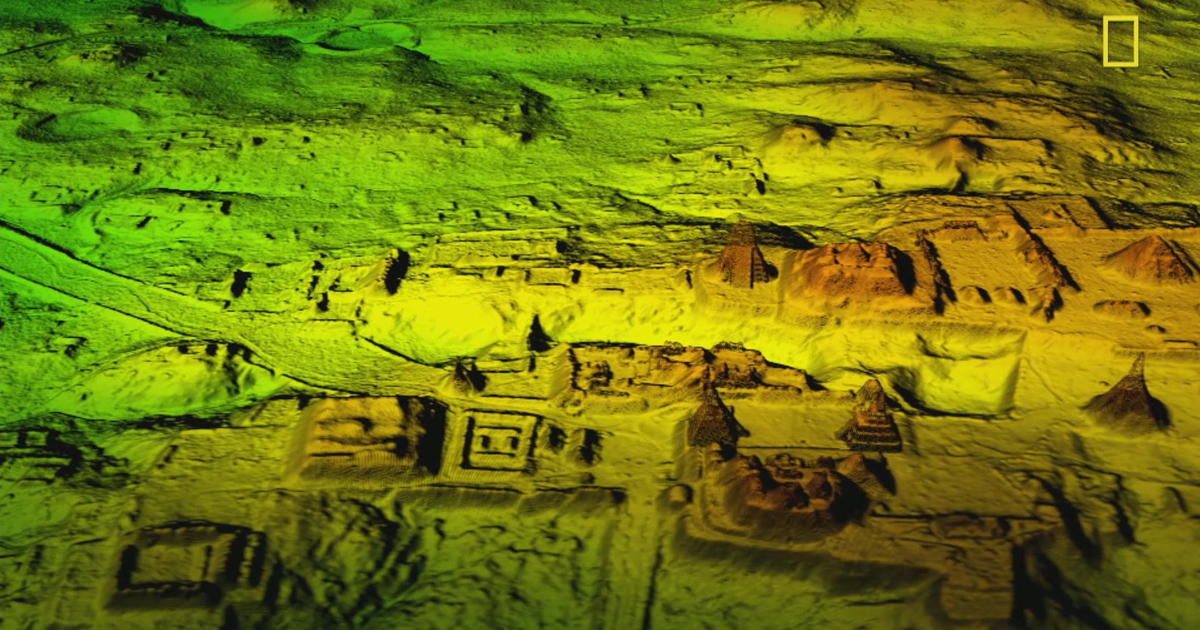This image, featuring the yellow National Geographic logo in the upper right corner, appears to be an aerial view of an ancient city, either Incan or Mayan in origin. The photo, possibly an artist's colorized rendering, depicts a detailed layout of various structures and temples, some reminiscent of pyramids. The landscape is hilly with sections that transition through green, yellow, and orange hues, suggesting different elevations or zones. The setting lacks any visible vegetation, indicating this might be a model or an artistic reconstruction showing how the city looked before natural decay. Old ruins and square foundations are visible, adding to the intricate depiction of what could be an impressive archaeological site, possibly even captured with an underwater photography technique for heightened effect. The multifaceted terrain also includes identifiable mounts and varied terrain depths.